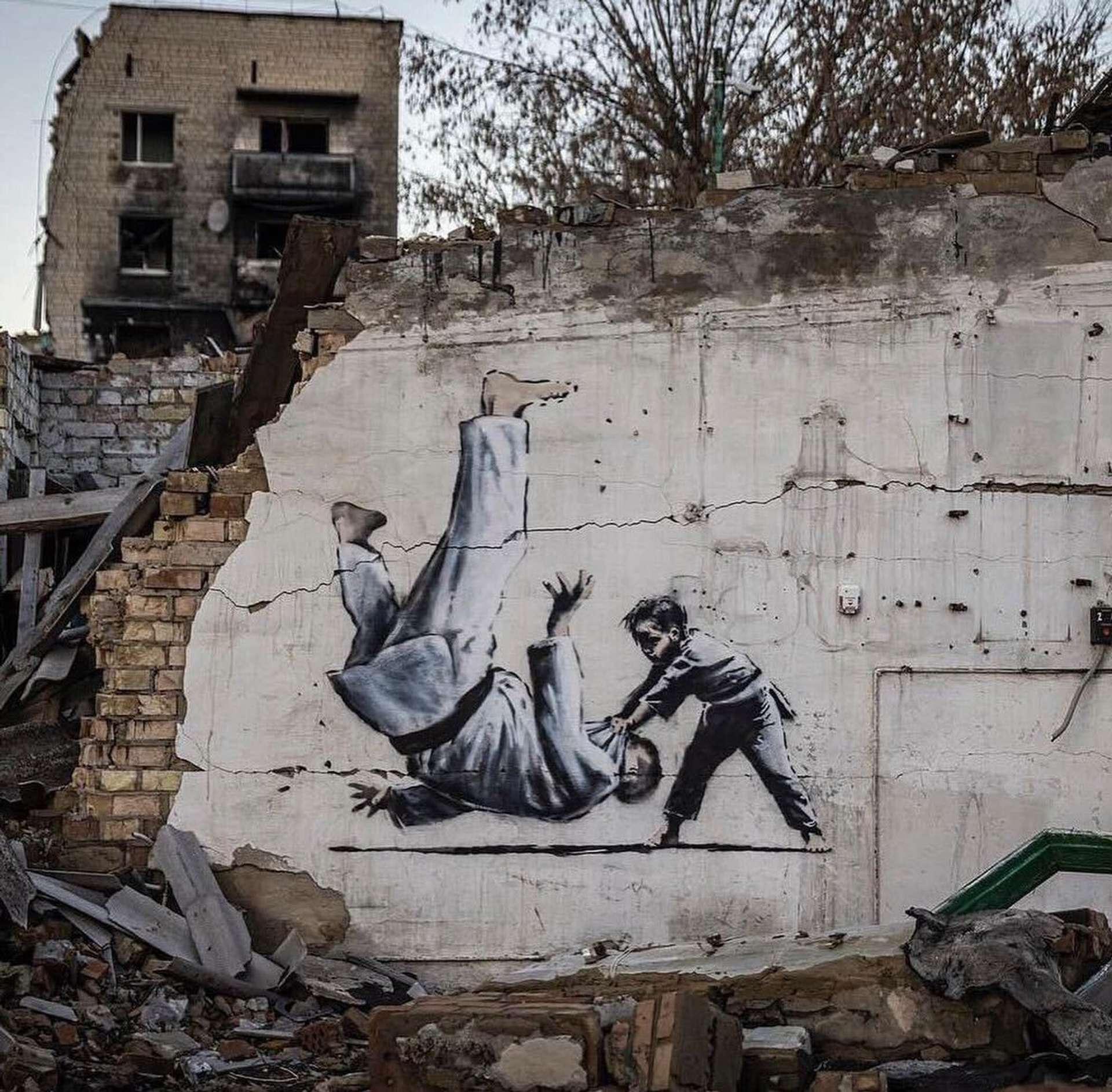The photograph captures a striking mural set against a backdrop of urban decay. The mural, painted on a crumbling brick wall, depicts a dramatic judo match between a small boy and an adult man. Both figures, who have fair complexions, are dressed in traditional white martial arts gis with black belts. The boy is caught in the act of performing a powerful throw, lifting the man by his shirt just as the man is about to hit the ground. This scene is vividly detailed and stands out amidst the surrounding ruins. The wall itself is severely damaged, with broken bricks, large cracks, and debris scattered around. In the background, there is a larger, decrepit building with extensive smoke damage, hanging wires, and remnants of a chimney or other structural elements lying on the ground. A tree rises behind the wall, adding to the sense of decay and abandonment that pervades the area. The vibrant mural contrasts sharply with the deteriorating buildings and rubble, adding a dynamic element to the otherwise bleak environment.